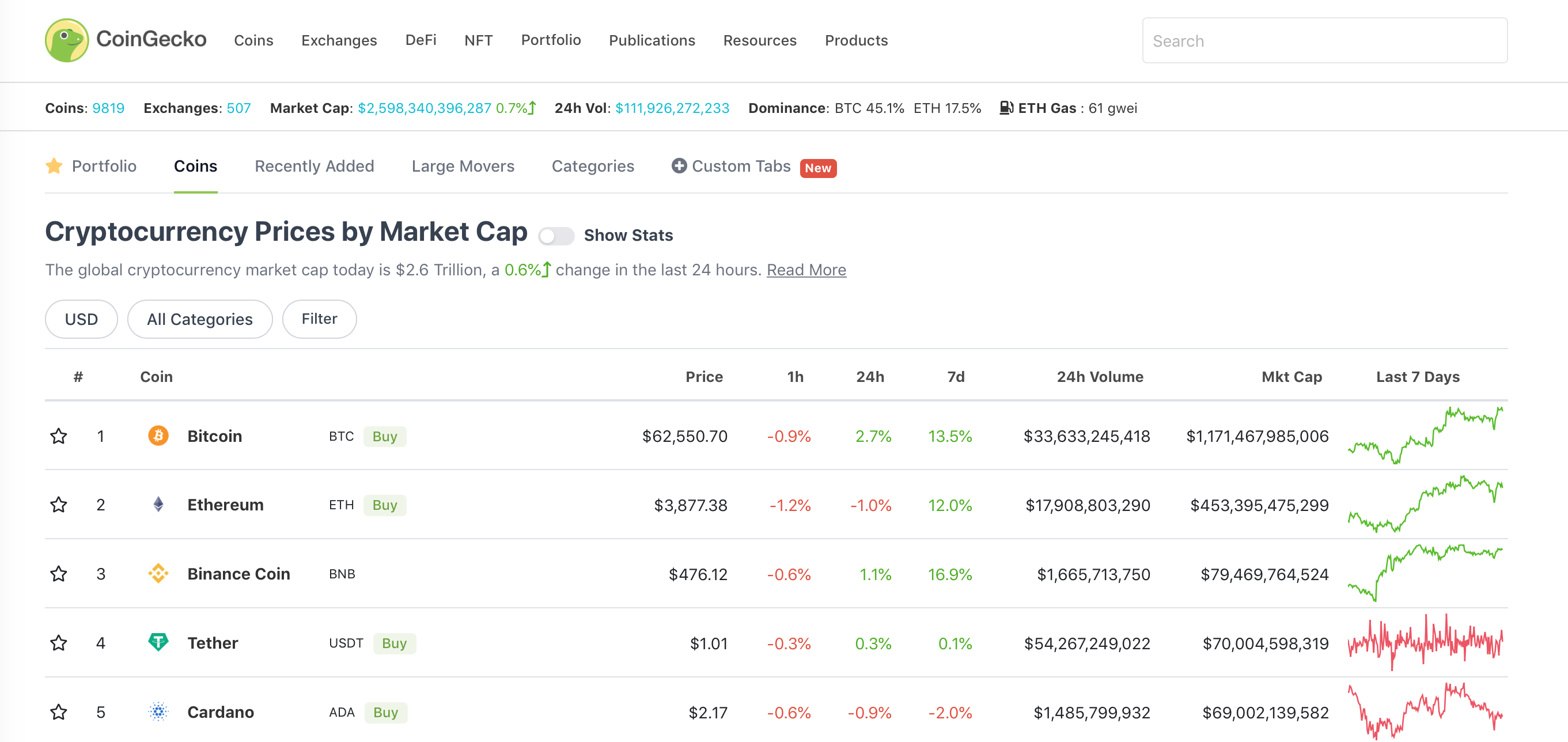**Descriptive Caption:**

This screenshot captures the homepage of CoinGecko. In the upper left corner, a profile picture features a bright yellow background with a cartoon green gecko facing right, adjacent to the "CoinGecko" logo in black letters. Adjacent to the logo, various menu options are listed: Coins, Exchanges, DeFi, NFT, Portfolio, Publications, Resources, and Products. 

On the upper right-hand side of the page, a search bar is prominently displayed. Below this, an information bar provides key cryptocurrency statistics: "Coins: 9,819," "Exchanges: 507," "Market Cap: $2,598,340,396,287," showing a 0.7% increase with an upward arrow, "24-hour Volume: $111,926,272,233," and "Dominance: BTC 45.1%, ETH 17.5%." Nearby, a gas pump emoji is shown with the text "ETH Gas: 61 GWEI."

The subsequent line features a yellow star at the left edge followed by "Portfolio." The "Coins" section is underlined in green, and additional tabs include "Recently Added," "Large Movers," "Categories," and "Custom Tabs," the latter marked with a plus symbol and a "NEW" red banner. 

A header then states, "Cryptocurrency Prices by Market Cap," along with an off switch for additional stat toggles and a "Show Stats" button. The following line reads, "The global cryptocurrency market cap today is $2.6 trillion," displaying a 0.6% increase from the last 24 hours with an upward arrow, followed by a "read more" link.

The main content consists of a detailed list of cryptocurrency entries and their respective graphs, arranged in five horizontal lines down the page.